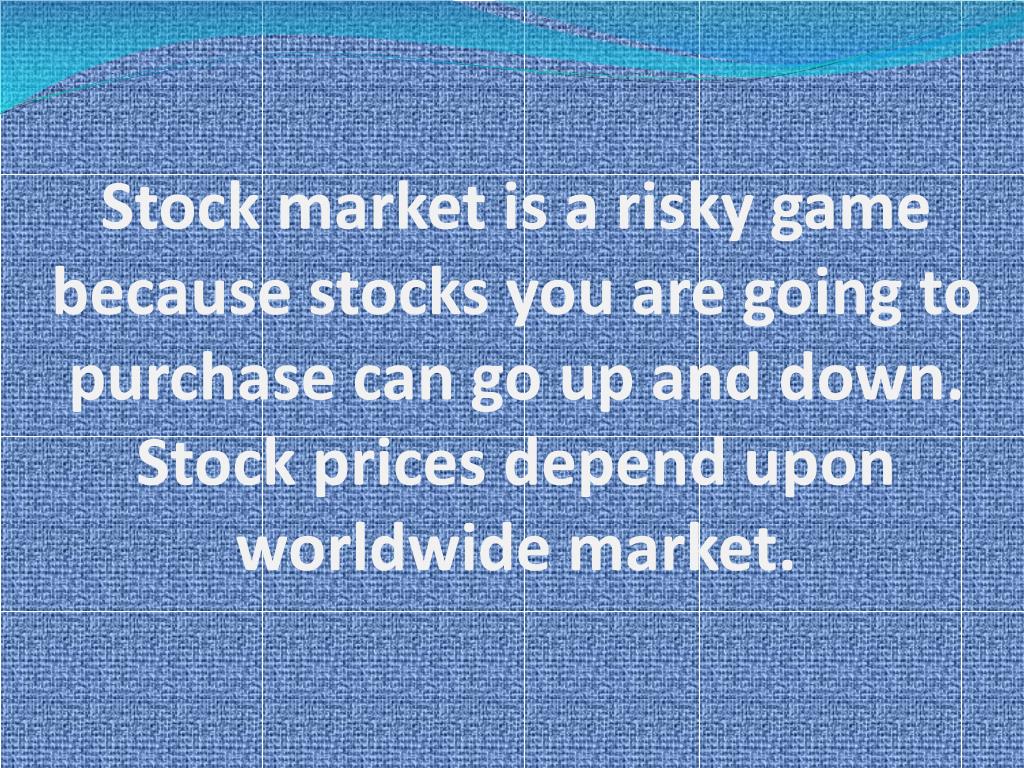The image features a bold text statement in white sans-serif lettering against a blue background with a nuanced design. The text reads: "Stock market is a risky game because stocks you are going to purchase can go up and down. Stock prices depend upon worldwide market." The grammar is not correct, but the statement emphasizes the volatility of the stock market. The background features a subtle grid pattern comprised of very thin white lines, both vertical and horizontal, creating a series of evenly spaced squares. A distinctive, lighter turquoise wave design adorns the top of the image, adding a graphical element that overlays the blue, fabric-like texture visible beneath. The primary focus of the image is the text, which is centrally positioned, dominating the visual space. The grid lines are mainly at the top where the text begins and just below where it ends, adding structure to the overall design. The combination of white and varying shades of blue, with the wavy turquoise header, provides a visual metaphor for the unpredictable nature of the stock market.